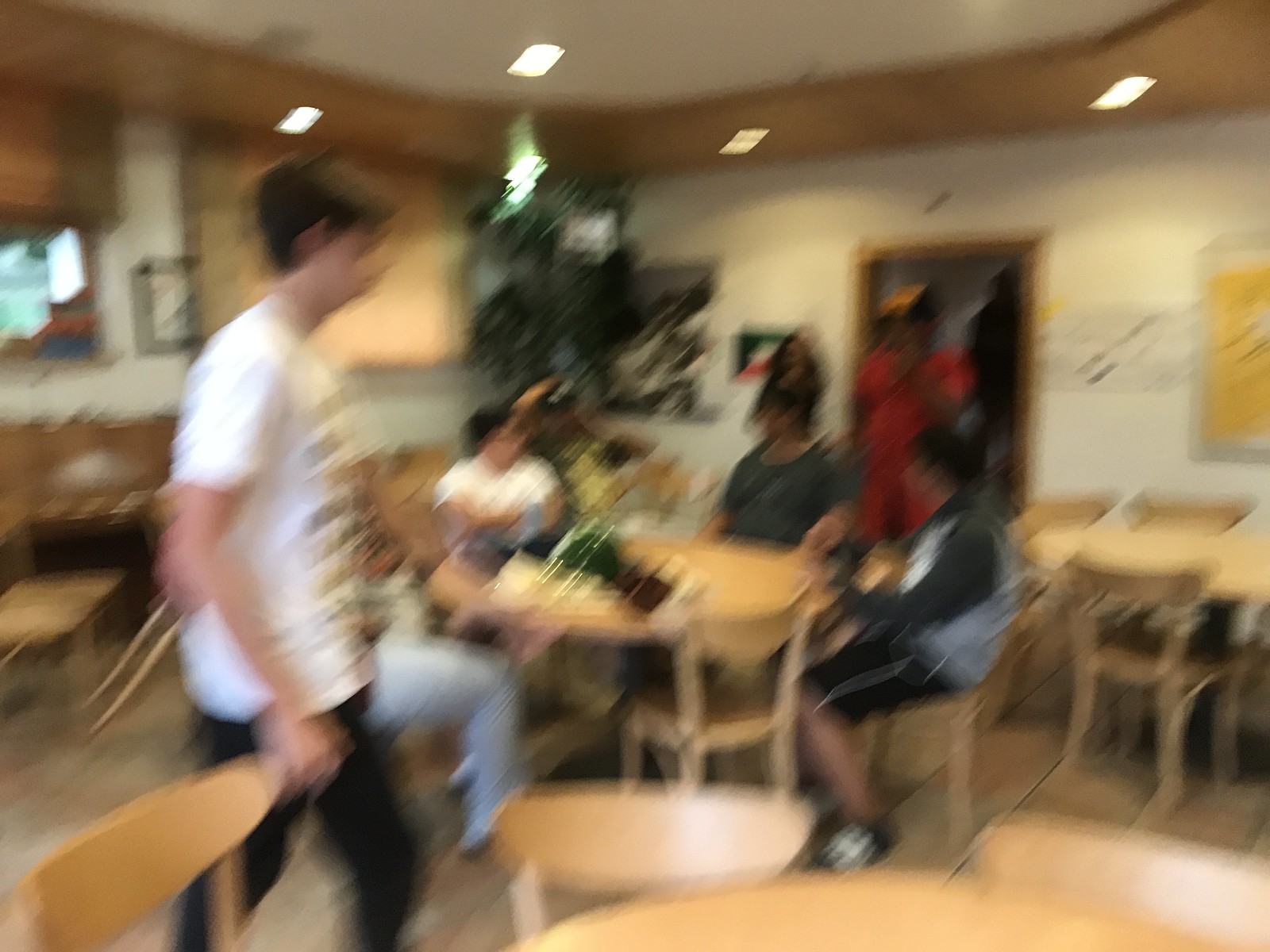The image, though blurry, captures a lively scene with eight people in a room furnished with wooden tables and chairs. On the left side, a person is seen walking behind a wooden chair. At the center of the image, three individuals are seated directly at a table, although only the right leg of one person is visible. Among the others, one individual is noticeable in a gray shirt, while another is dressed in a gray and black top with black shorts. To the right, a person stands in a doorway, distinguished by their red attire, next to another individual with long, dark hair wearing a black shirt. Additionally, two more people are seated near the table but not at it; one wears a white shirt, and the other is identifiable by a black cap. In the background, a green plant occupies the far corner, and various paintings adorn the walls, adding to the room's decor.